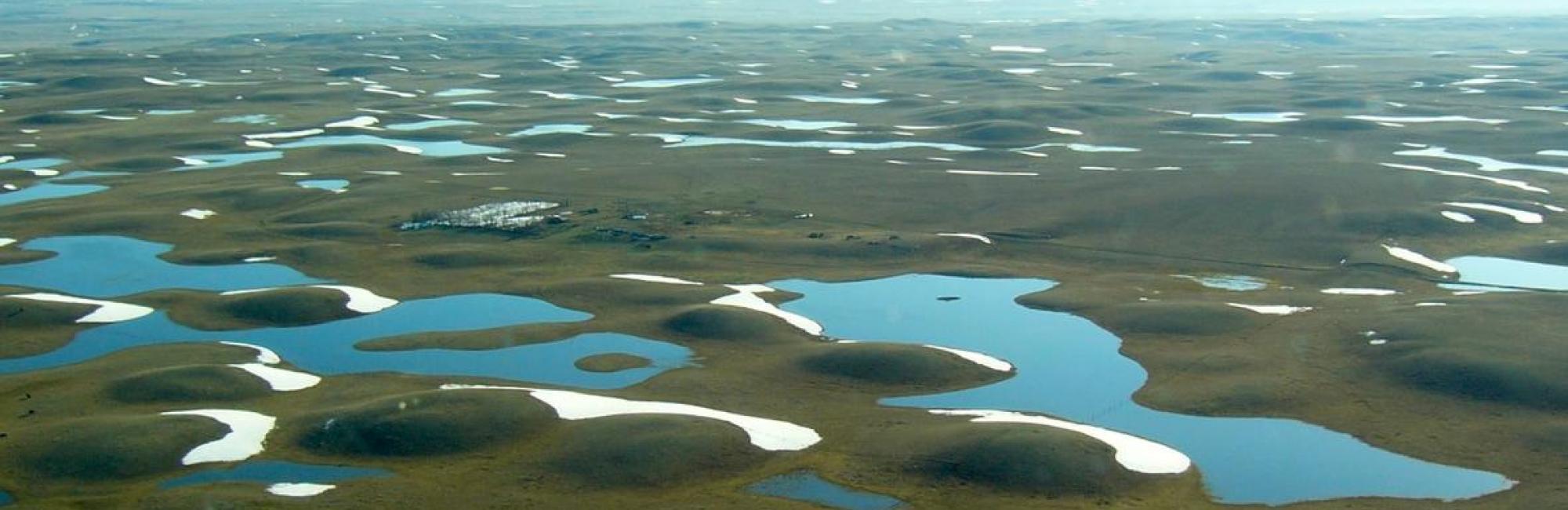This horizontal, aerial photograph captures a vast, moisture-rich landscape characterized by numerous small, snow-capped hills and mounds spread across the scene. The snow appears to be melting, creating large areas of pooled water that intersperse the greenish, mossy ground, suggesting a highly saturated environment. The image spans a considerable distance, reaching all the way to the horizon. 

In the center of the composition, there appears to be a cluster of buildings or a remote station, possibly a power station, accessible by a road cutting through the terrain. These man-made structures add interest and contrast to the otherwise natural setting. Raised rock formations contribute to the moon-like surface, dotted with pools of water and occasional greenery. The sky is likely blue, providing a serene backdrop to this intriguing mixture of natural and human elements.